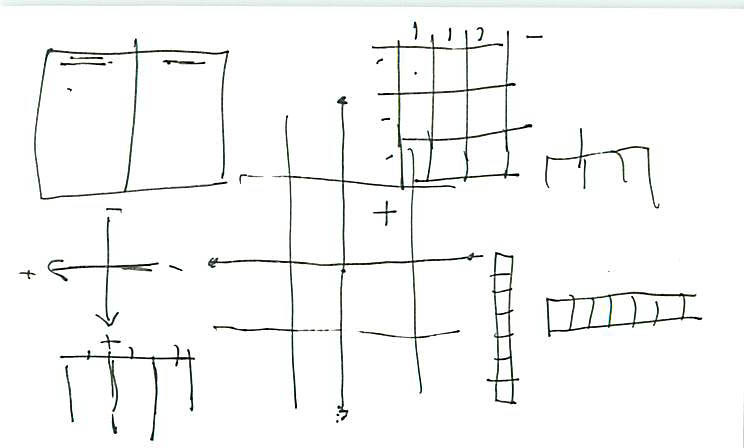Detailed Description: 

This image displays a complex, hand-drawn diagram rendered entirely in black ink on a white sheet of paper. The diagram is segmented into various sections with distinct symbols and structures.

In the top left corner, it begins with a square that is bisected vertically by a single line. Additionally, there are two short lines originating from the top left corner, and another from the top right corner of the square. 

Adjacent to this, in the top right section, a meticulously drawn grid composed of three rows is observed. Each section of this grid appears to be numbered, likely with ones above each block.

Moving further left, there's a plus-shaped symbol in the upper left corner. This symbol features an arrow pointing downwards and a small plus sign on its left side.

Beneath this, there is a section defined by a grid of lines. It comprises four vertical lines and four horizontal lines, with the horizontal line positioned at the top.

Near the center-right section of the page, a larger box is depicted, resembling a tic-tac-toe grid. It is divided by three vertical and three horizontal lines, with a distinct plus sign marked in the top right cell of this grid.

Finally, in the bottom right corner of the diagram, there's a representation of vertical and horizontal bars, reminiscent of graphs or charts. A single vertical and a single horizontal bar intersect, creating a foundational cross. Above this intersection, in the top right, there is a pitchfork-like drawing featuring a single horizontal line atop a box shape, from which four vertical lines extend downward.

This detailed depiction covers the entirety of the diagram, highlighting its complexity and varied symbolic elements.